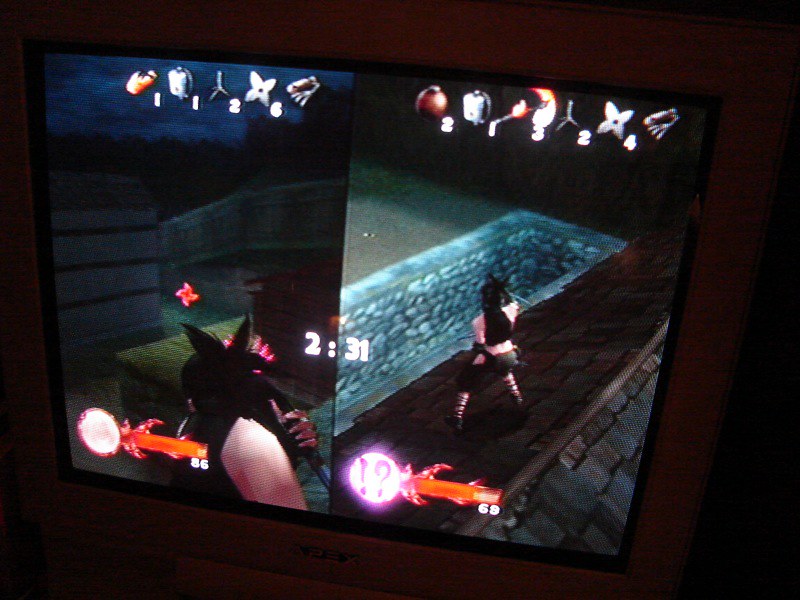The image depicts a television screen showcasing a third-person action video game, illuminated by dull red lighting. The screen is bordered by a silver frame, with a small logo and speakers positioned beneath it. At the center of the screen is a timer displayed in white, reading "2:31." The game interface includes various icons and numbers at the top—one side shows "1-1-2-6" and the other "2-1-3-2-4" in shades of brown, white, and orange. A power bar exists on each side of the screen: one reads 86 with a red ninja star-like symbol nearby, and the other reads 69 with a purple spot featuring an exclamation mark and question mark. The player character, a dark-haired warrior in a revealing black outfit, stands battle-ready before a stone pit. The life meter and weapon choices are arranged along the bottom of the screen.